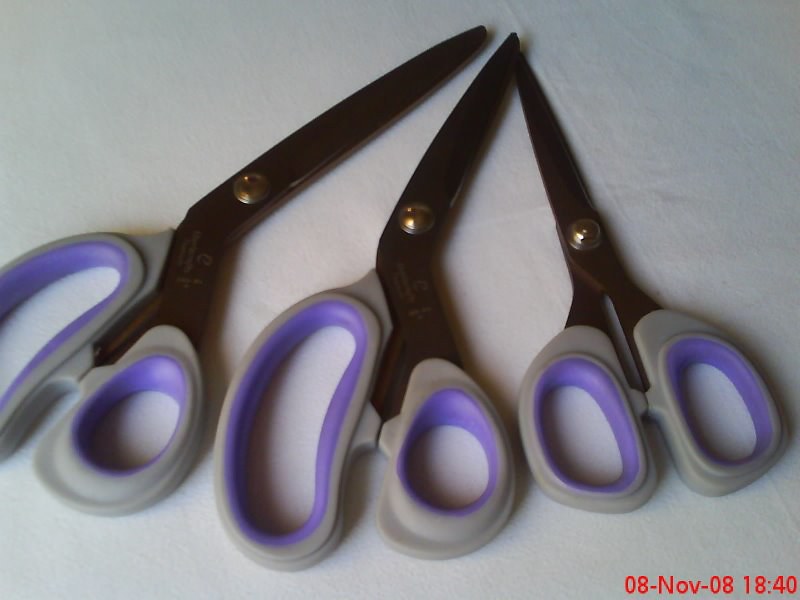The image shows three pairs of scissors arranged on a white tablecloth, forming a triangular shape with their handles spread out. Each pair of scissors features gray handles with a light purple interior and a brass-looking rivet at the center, which acts as a hinge. The scissors vary in size: the smallest is on the right, a medium-sized pair is in the middle, and a large pair is to the left. The larger scissors have long, pointed blades, and the handles are described as plastic for safety reasons. The photograph, which appears to be slightly fuzzy and taken digitally, includes a date code "08-NLV-08" and a timestamp "1840," suggesting it was taken in 2008. The handles are gray on the outside and violet on the inside, reinforcing a consistent design across the different sizes. The white fabric or tablecloth provides a neutral backdrop that highlights the scissors' details.